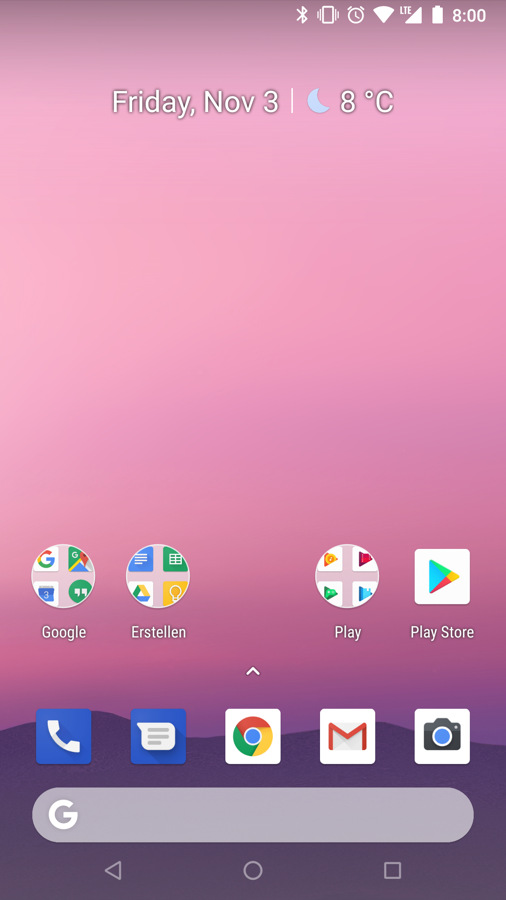The image showcases a mobile device or tablet displaying a web page with a serene and dreamy aesthetic. At the top of the screen, the date "Friday, November 3rd" is prominently displayed, followed by a quarter moon icon and the temperature reading of "8°C". The background is a soft light pink, gradually transitioning to a reddish hue, suggesting an early morning or late evening sky. The sky itself is clear, with no clouds in sight, offering a calm and uncluttered view.

As the scene extends downward, a subtle gradient of colors presents itself, beginning with a gray hilly area at the bottom that transitions into a delicate purple shade higher up. This picturesque background employs a mix of pinks and purples to capture the fleeting moments of dawn or dusk.

Overlaying this tranquil sky, the display mimics the home screen of a mobile device. At the bottom, a gray search bar with the Google "G" logo encourages quick searches. Above it, several app icons are neatly arranged in a row: classic symbols for phone, notes, Google or Chrome, mail, and camera. Just above these, three round icons denote apps like Google, a possible "Stellan" app, and the Play app, while the Play Store icon is distinctly encased in a square.

Overall, this beautifully detailed depiction harmoniously blends the utility of a modern mobile interface with the serene beauty of a twilight sky, creating a captivating and functional visual experience.